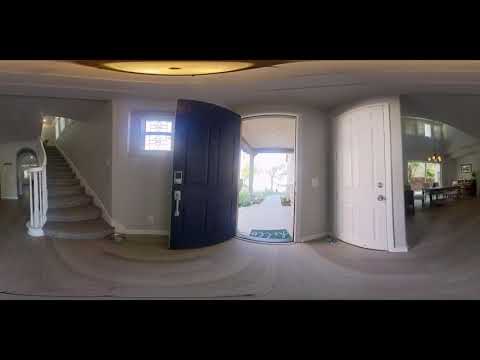The image depicts a well-lit entrance to a home, with a black front door featuring silver hardware at the center. The door is swung open, revealing a small porch outside. Directly to the left of the entrance, there's a small window and a staircase leading upstairs with a white banister and gray carpeting. A mat is placed at the doorway. To the right of the front door, there's another white door also with silver hardware, and an opening leading to a room containing a large window, silhouettes of furniture, and potentially a view towards the backyard or patio. The beige carpeted floor and cream-colored walls give the space a cozy feel, and a large light fixture illuminates the entryway. The overall wide-angle perspective shows the expansive living room to the right with high walls, chairs, a table, and a picture on the wall.